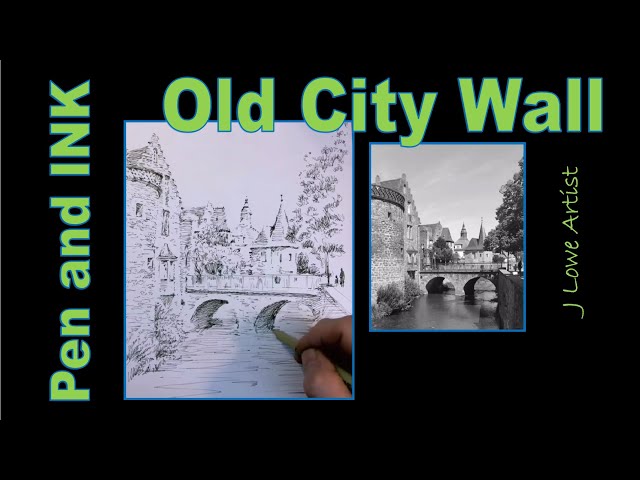Against a black background, the image prominently features the text "Pen and Ink" in green, displayed sideways from the bottom to the top. At the top of the image, the text "Old City Wall" appears in green, accompanied by the name "J. Lowe, Artist" on the right side, also displayed sideways. 

The central part of the image showcases two depictions of a detailed pencil sketch. On the left side, a larger image features a man sketching an old-timey city scene with a bridge, waterway, steeples, and buildings— all rendered in black and white. This sketch includes details like a flowing river beneath the bridge and various architectural elements suggesting a historic cityscape.

On the right side, a smaller, more detailed version of the same scene is shown. The second image represents the progression of the drawing, capturing even finer details and greater clarity, including additional architectural features and a prominent tree.

This dual depiction contrasts the initial sketch with its more refined state, offering viewers a visual progression of J. Lowe's intricate "Pen and Ink" artistic process, illustrating the meticulous efforts in creating the old city scenery.